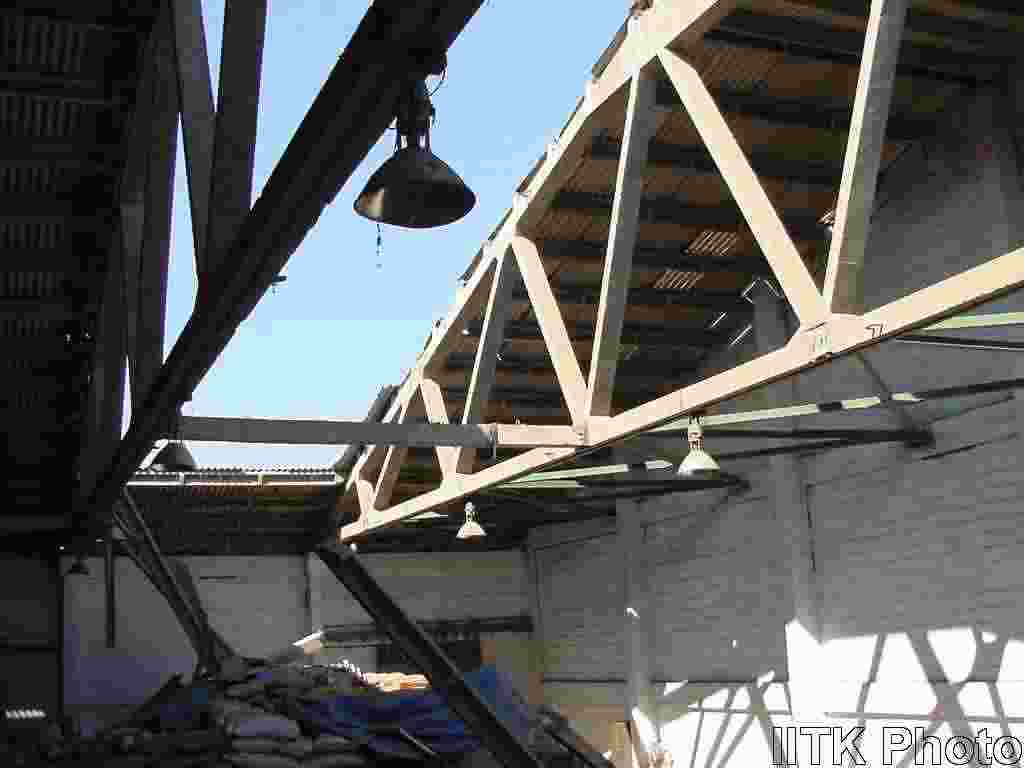The image depicts the interior of what appears to be an abandoned or partially demolished industrial building, potentially a factory. The roof has a domed shape and features a significant collapsed section through which the bright blue sky is visible, allowing sunlight to stream in. The remaining roof trusses, made of metal with a reddish hue and a white tint, support the undamaged sections. The underside of the roof has a yellowish-orange color. The white brick walls wrap around the area, standing out despite the pixelation of the image.

A criss-cross pattern of metal beams spans the ceiling, from which several green metal lights are suspended. A rectangular opening in the roof showcases the open air, hinting at structural failure or deliberate demolition efforts. Below the collapsed section, piles of debris and what appear to be sandbags are scattered on the ground. Distinctive features include a cone-shaped bell hanging from one of the light-colored wood beams. The bottom right corner of the image contains a black border with the text "IITK photo."

Together, these details suggest the building is undergoing demolition or cleanup, capturing a moment where natural elements and remnants of the structure coexist in a state of transition.